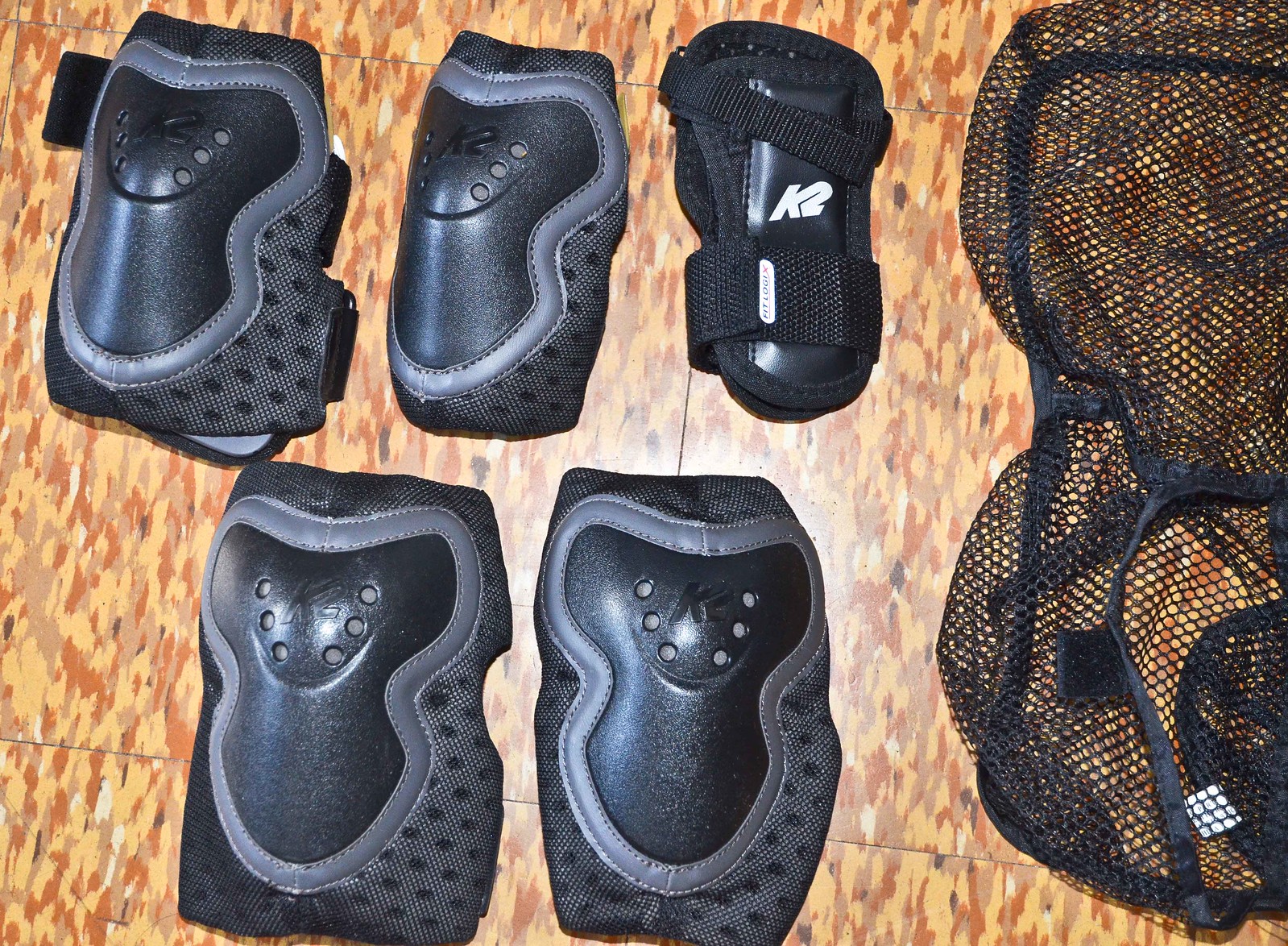A top-down photograph showcases protective sports gear, including knee pads, elbow pads, and a wrist brace, all arranged on a light brown, tile-patterned floor with dark brown and orange blotches. In the upper left are two identical elbow pads featuring black straps with darker splotches, a central black protective cup outlined in gray, and visible black straps extending from behind. The knee pads, twice the size of the elbow pads, are positioned below and slightly to the left. These knee pads also have a black plastic shell with six ventilation holes and a central K2 logo, outlined in gray fabric. A black wrist brace with a white K2 logo is beneath two elbow pads. On the far right, a black netted bag with black borders stretches from the top to the bottom of the image, likely used for carrying the protective gear.